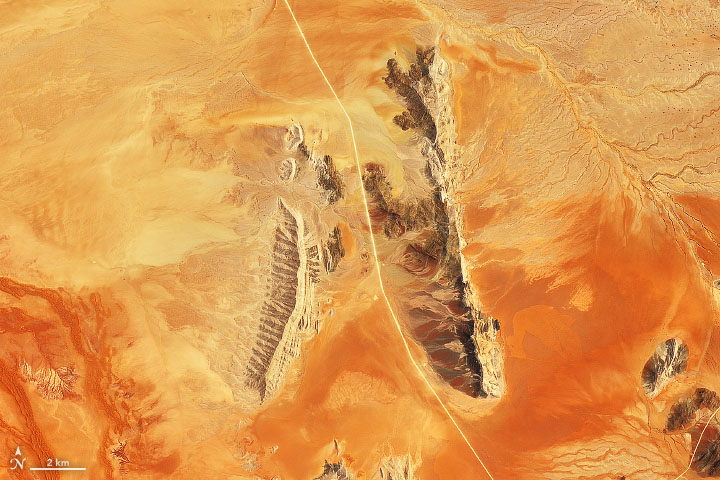This image captures an overhead, landscape-oriented view resembling satellite imagery of a desert terrain. The composition predominantly features a vast expanse of reddish-brown sand interspersed with darker brown patches of land, suggesting rocky outcrops or small mountain ridges. Notably, a light-colored road, curving slightly and running vertically down the center, divides the scene. Towards the left of this road, smaller rock formations and a lighter brown mountain ridge are visible, while to the right, larger reddish rocks and a more prominent ridge can be discerned. Additionally, in the bottom left corner of the image, a directional key is present showing an 'N' with an arrow pointing upwards, indicating North, alongside a horizontal line labeled '2 km', which provides scale. Near the bottom right, some lines spread out in various directions, potentially hinting at a river or creek cutting through the arid landscape, contributing to the intricate veiny patterns on the desert floor. The overall coloration of the image varies, with lighter sandy hues at the top transitioning into deeper reddish tones toward the bottom, evoking a sense of a sun-drenched, fiery desertscape.